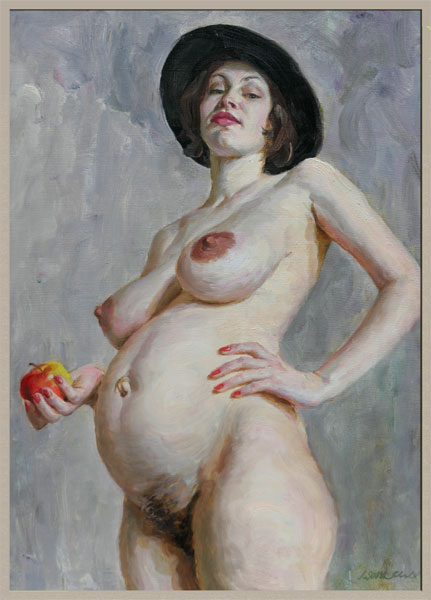This detailed painting by Victor Liapkalo, titled "Kate, Wear a Hat" and created in 1998, captures a nude, pregnant woman standing confidently and facing the audience. The painting, done in an oil-on-canvas, kitsch style, features the woman with short brown bobbed hair under a wide-brimmed black hat. Her left hand rests on her hip, with her elbow crooked, displaying nails painted brightly red. Her right hand holds a red and green apple. She has very large breasts with prominent nipples, a wide belly with an outie belly button, and a linea nigra extending from beneath her belly button to her ribcage. Her plump, pink lips give her a subtle, subtle smile as she gazes directly at the camera against a varying gray background. The frame surrounding the painting is an ivory-gray color, matching her skin tone. At the bottom right, there's an illegible signature from the artist.